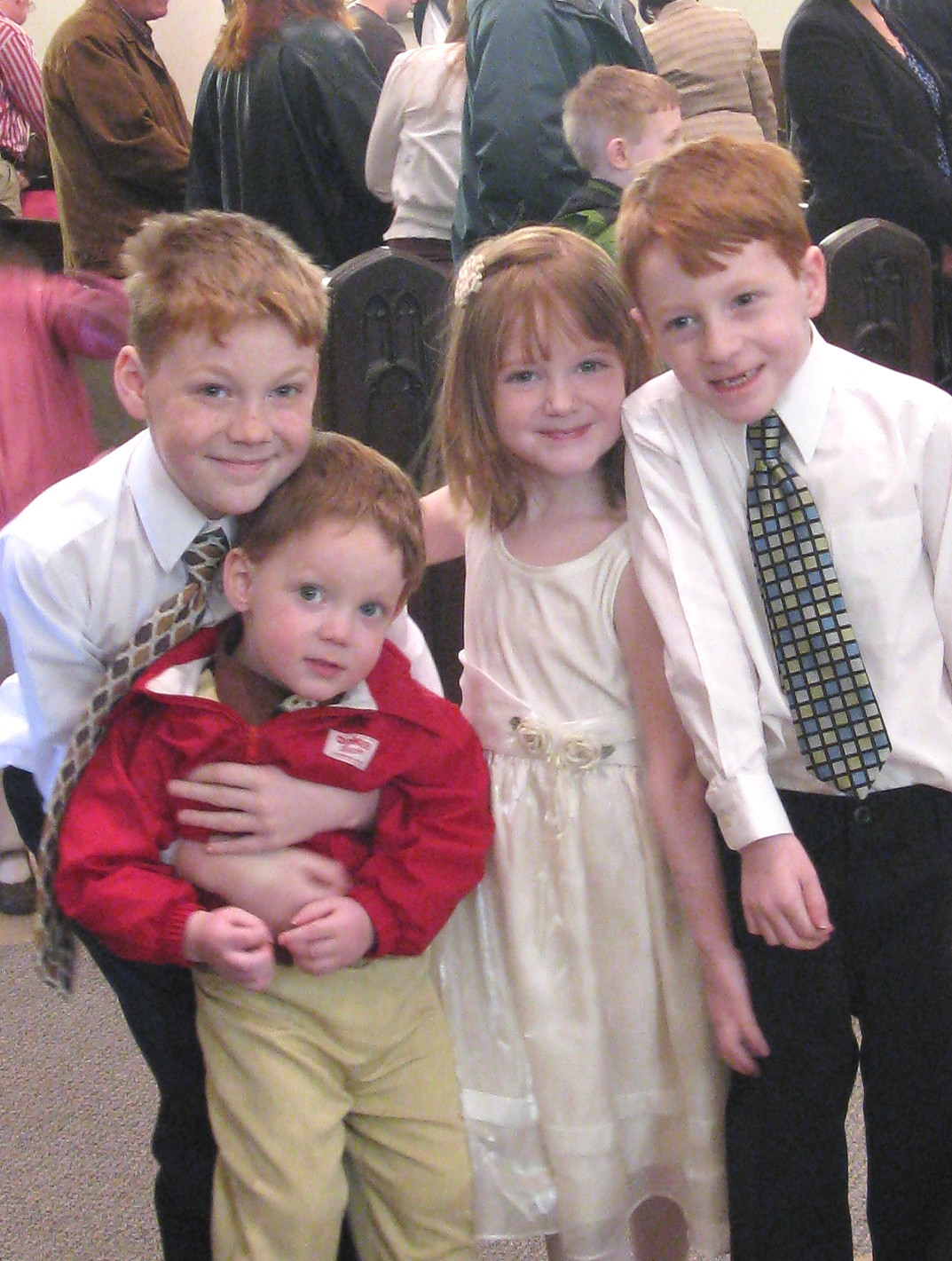This detailed photograph captures a special occasion, likely taking place in a church, as evidenced by the brown pews and the people seated in the background. Amongst the people, a woman in a black choir robe can be observed. The floor is carpeted in light tan. The focal point is four red-haired children, who appear to be siblings, dressed in their Sunday best. In the foreground, one boy, who seems to be the oldest, is dressed in black pants, a white long-sleeve shirt, and a checkered tie. He is holding the youngest child, a toddler, who is outfitted in tan khaki pants, a brown shirt, and a red zip-up jacket. Another older boy similarly wears black pants, a white shirt, and a patterned tie. The little girl among them is adorned in an ivory-colored dress with lace at the bottom, a belt featuring roses, and a white bow in her hair. They stand on the plush, light carpeted floor, creating a heartwarming familial scene amidst the backdrop of a formal event such as a wedding or baptism.